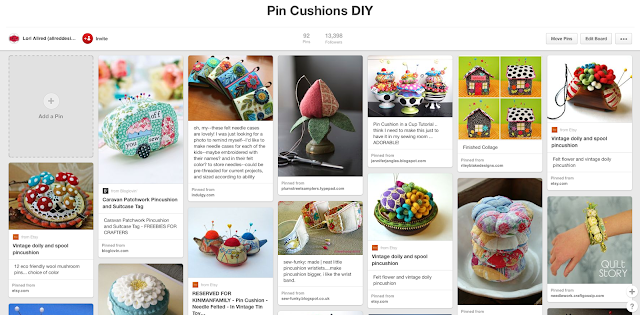A website dedicated to DIY projects and pincushions features a grid layout with numerous squares showcasing various images. The first square, which is gray, prompts users to "Add a Pen". Following this, several vertically-oriented rectangles display images with detailed descriptions. 

The first image resembles a rolling suitcase covered in numerous pushpins, giving it a quirky and functional appeal. The second image features a collection of miniature books, meticulously arranged to capture the charm of a tiny library. The third image showcases a vase with a plant or flower, creatively repurposed to hold a pen within the bloom. The fourth image depicts a delectable dessert setup, possibly cake, served in three bowls, adding a touch of culinary delight to the assortment of visual content.